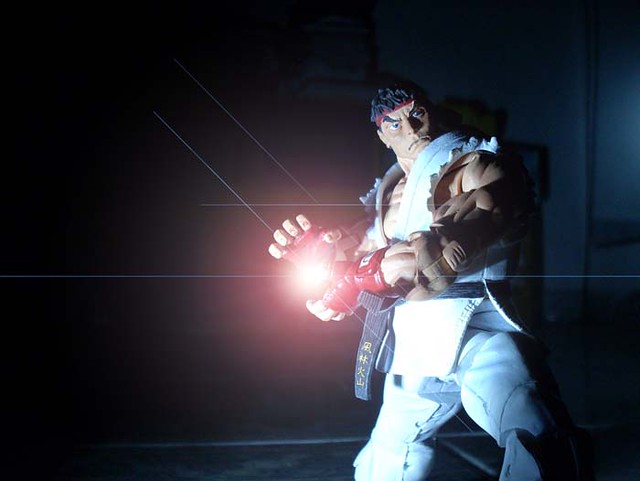This wide rectangular image features a digitally recreated, highly detailed action figure set against a dark background that fades especially deep on the left side. The figure, positioned slightly right of center, faces left and showcases a body with light tan skin and impressively large, muscular arms. These arms, adorned with red, fingerless, soft-looking gloves, are extended leftward, holding a brilliant orb of light that seems to be the sole light source, illuminating the figure amidst the darkness. The figure boasts an intense facial expression with large, dark eyes, spiky black hair held by a red headband, and a frown etched across its face. Sharp, bent eyebrows highlight its anger. It wears a white, tank top-like shirt, revealing a powerful chest, and has white trousers paired with a black belt adorned with yellow Chinese characters. Contributing to the dark, dramatic aesthetic are thin white lines and rays emanating from the orb, crossing the background diagonally and horizontally, adding a dynamic, otherworldly atmosphere to the scene.